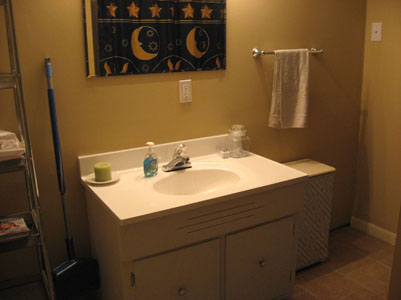The image portrays a typical bathroom interior with a cozy and organized setup. The walls are painted a soothing beige, setting a warm tone for the room. Dominating the central wall is what appears to be a medicine cabinet or a mirror, reflecting a creative shower curtain adorned with whimsical designs of beige moons and a horizontal line of stars against a black background, matching the wall color.

To the right of this mirror or tapestry is a neatly folded white towel hanging on a towel rack. Beneath the towel rack sits a white laundry hamper, maintaining the room's clean aesthetic. Directly below the mirror or wall decoration is a wide, single sink with ample storage space. The cabinetry features two white doors with central knob handles, adding functional elegance.

On the sink's surface, there is a green candle placed on a white saucer to the left, providing a touch of tranquility. Adjacent to the candle, a chrome faucet is flanked by a hand soap dispenser. On the right side of the sink, a glass container offers additional storage, though its contents are not discernible.

Further to the left of the sink and cabinetry, a navy blue broom leans against the wall, next to a brown wooden ladder shelving unit that adds a rustic charm and extra storage options. The floor is covered in beige-ish brown tiles, tying the room's color scheme together harmoniously. There are no text elements within the image, allowing the focus to remain on the bathroom's inviting and functional design.